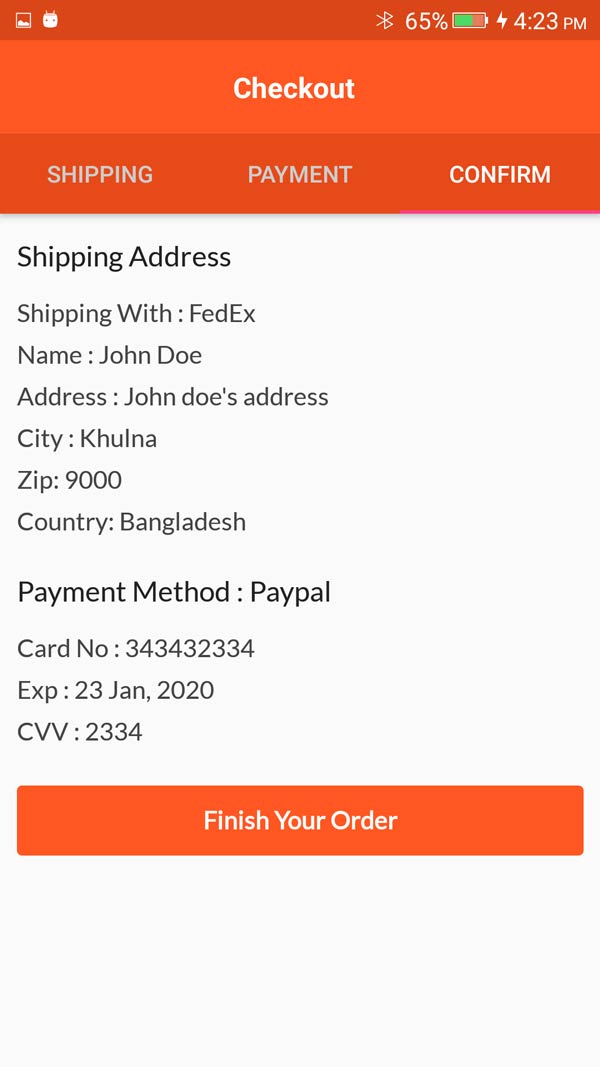In the screenshot of a FedEx order displayed on a mobile device, the screen features a predominantly orange and white theme. It's evident that the mobile device's battery is currently charging, showing a 65% charge level. Bluetooth is enabled, and the time displayed is 4:23 p.m. 

At the top of the screen, the word "Checkout" is prominently displayed in white font on a lighter orange banner. Below it, three steps are outlined—Shipping, Payment, and Confirm—on a darker orange banner. 

The shipping details show the recipient’s name as John Doe, with the address listed as John Doe's address in the city of Kulna, zip code 9000, in Bangladesh. The shipping method chosen is FedEx. 

For payment, the method selected is PayPal, displaying a partially obscured card number (343-432-334), with an expiration date of January 23, 2020, and a CVV of 2334. 

At the bottom of the screen, there's a prominent orange button labeled "Finish Your Order," inviting the user to complete the transaction.